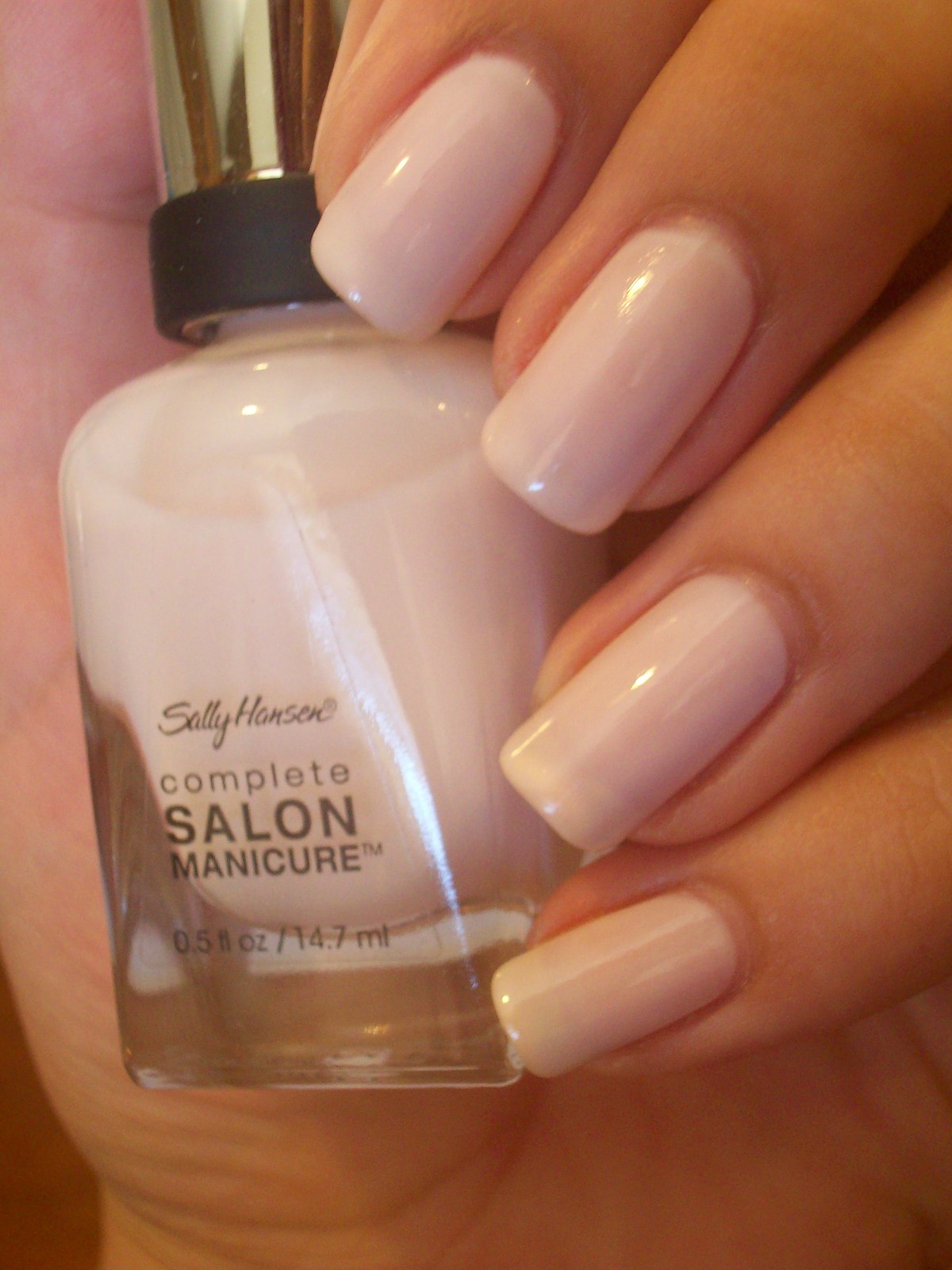The photograph is a close-up shot focusing on a woman's hand, showcasing her freshly manicured nails. She holds a clear bottle of Sally Hansen Complete Salon Manicure nail polish, with a gold and black screw-on cap. The polish inside the bottle and on her nails is a light pink hue, perfectly matching. Her nails are fairly long and have a straight, not rounded shape, with a meticulous manicure that accentuates her clean cuticles. The text on the bottle reads "Sally Hansen Complete Salon Manicure 0.5 FL OZ / 14.7 ML." While all her fingers are visible, the thumb is not in the frame. The overall composition highlights the elegance and refinement of both the manicure and the nail polish product.